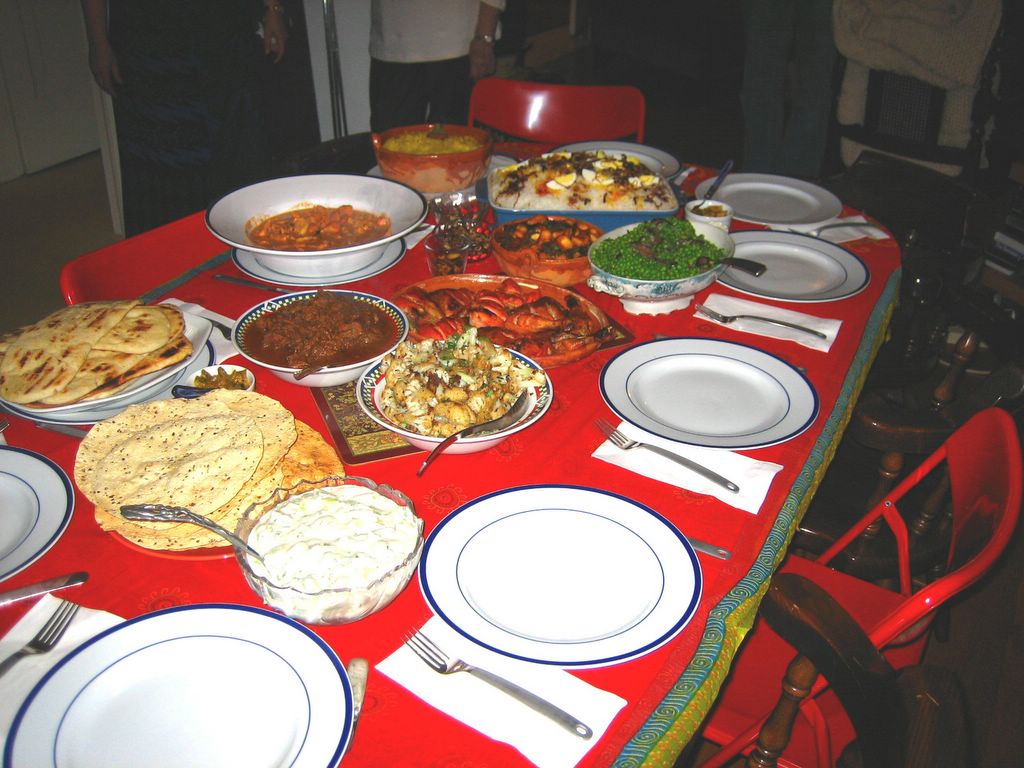The image captures a vibrant dining setting within someone's home. A table is elegantly set with blue and white plates arranged around the right perimeter, each complemented by a white napkin with a fork placed to its left. The table is draped in a red cloth, with an array of dishes featuring various types of food positioned centrally and to the left. Among the culinary offerings are a brown stew, bread, peas, beans, tortillas, a bowl of white sauce, possibly some taco ingredients, and a dish that could be either a cake or a salad in an oblong blue dish. Additionally, there appears to be a bowl of potatoes and another with vegetable soup. A white styrofoam cup can be observed on the right, adding to the informal, homey atmosphere. On the right side, several red folding chairs are pulled up to the table, ready for the gathering. At the top of the image, a row of people stands behind the table, but the photo only captures their torsos, missing their heads and legs. This scene is set for a meal, bustling with an array of foods and the warm anticipation of a shared dining experience.